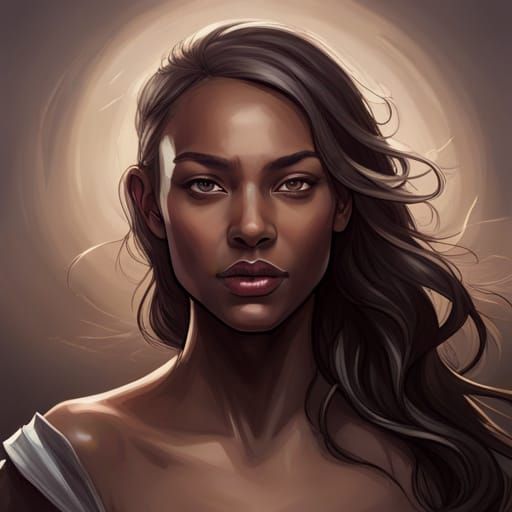The image features a woman with a serious, intense gaze, her long, wavy dark brown hair cascading over to the right side, revealing most of her ear on the left. Her complexion is a rich, bronze tone that blends seamlessly with the background, which has a bronze hue with a gradient fade to lighter shades, accented by a swirling white light reminiscent of a halo or sunburst behind her head. She wears a light gray, off-the-shoulder top that falls slightly off her right shoulder (the left side of the image). Her lips are adorned with reddish lipstick, adding a pop of color against her bronzed skin. The portrait captures her from just above her head to slightly below her chest area, emphasizing her serious demeanor and cohesive, warm color palette that dominates the frame.